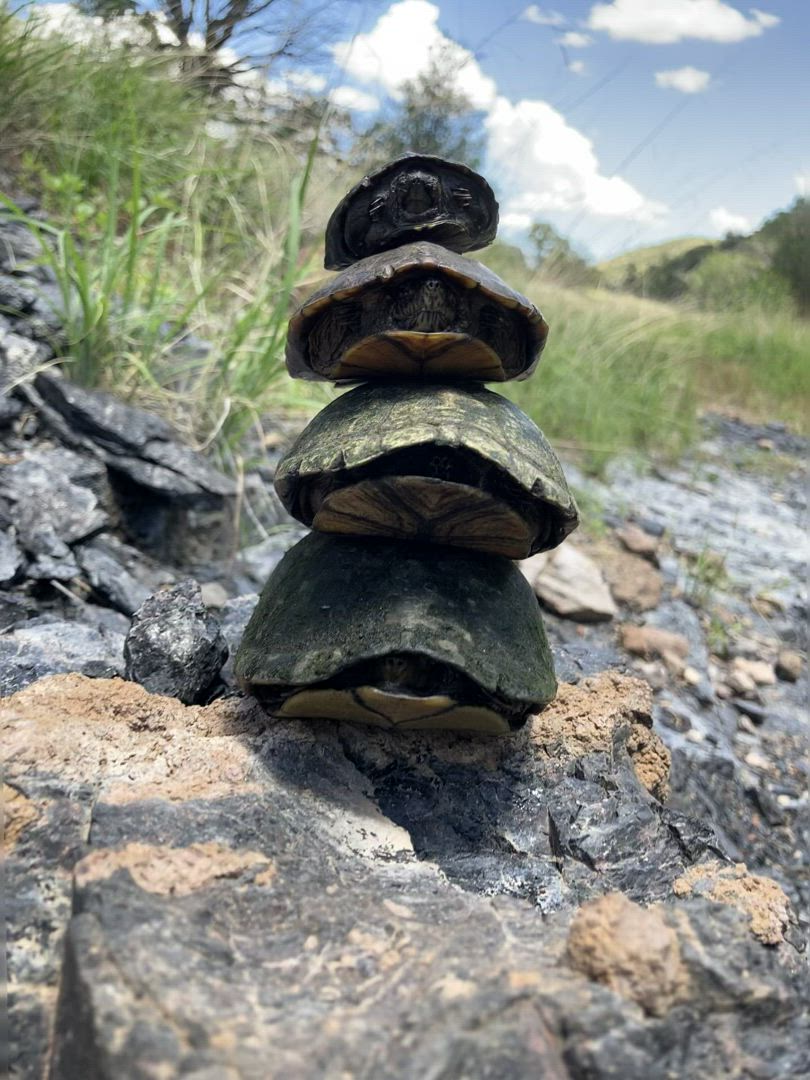This is a detailed outdoor photograph of a picturesque scene on a sunny day featuring a unique stack of four turtles on a large, dark gray rock adorned with brown dirt and some patches of moss. In the foreground, a big turtle with a green shell and a tan underside forms the base of the stack, laying firmly against the rocky surface. On top of this large turtle, there is a slightly smaller turtle, also with a similar green shell, though its head and body are not visible as it is tucked deep inside its shell. Continuing upward, the third turtle is somewhat smaller and has its head peeking out slightly, providing a glimpse of life amidst the stack. The smallest, darkest (almost black) turtle perches at the very top, its head sticking out more prominently.

Surrounding the rock, the landscape transitions into a lush bed of healthy green grass interspersed with tall weeds and small rocks. The scene extends into the background where the grassy area meets some distant trees, completing the natural setting. Above, the sky is a vibrant blue, dotted with fluffy white clouds, framing this captivating snapshot of turtle behavior and their serene habitat.